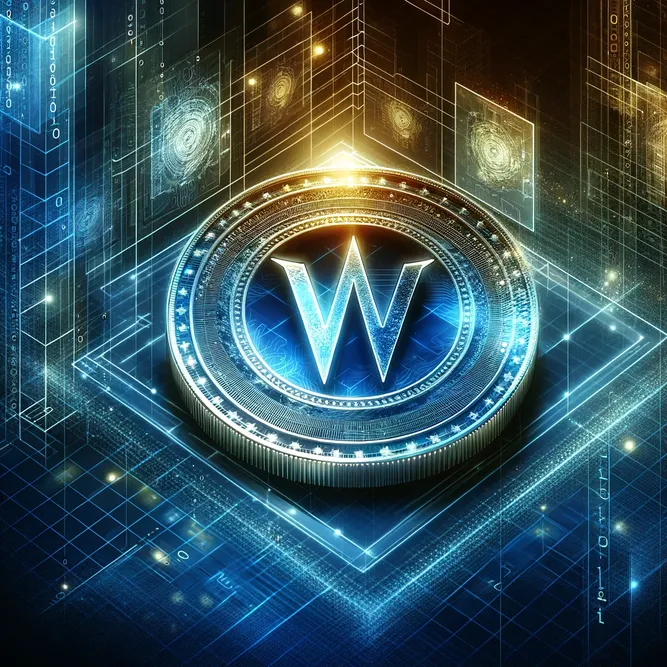The image is a vibrant, computer-generated artwork dominated by a central coin-like structure featuring a prominent letter "W." This coin is set within multiple concentric circles, giving it a 3D, reeded edge appearance. The letter "W" is outlined in a fiery, gold-like font, adding to its intricate design. The background is a mix of dark blue, light blue, and hints of teal, with a complex, futuristic architectural layout that resembles a high-tech chipset board with intersecting lines and structures.

The image is illuminated by a yellow light that permeates through the top portion, casting a subtle glow. Surrounding the central circle are multiple smaller squares containing swirl patterns, some resembling galaxies. The top left corner features indecipherable writing, and additional text at the bottom appears to spell "L-O-L-O-L-E-T." Towards the lower part of the image, the colors transition to darker blues with specks of gold.

Overall, the picture combines elements of 3D modeling, architectural design, and futuristic aesthetics, creating a captivating and detailed representation of a digital coin in a high-tech, abstract environment.